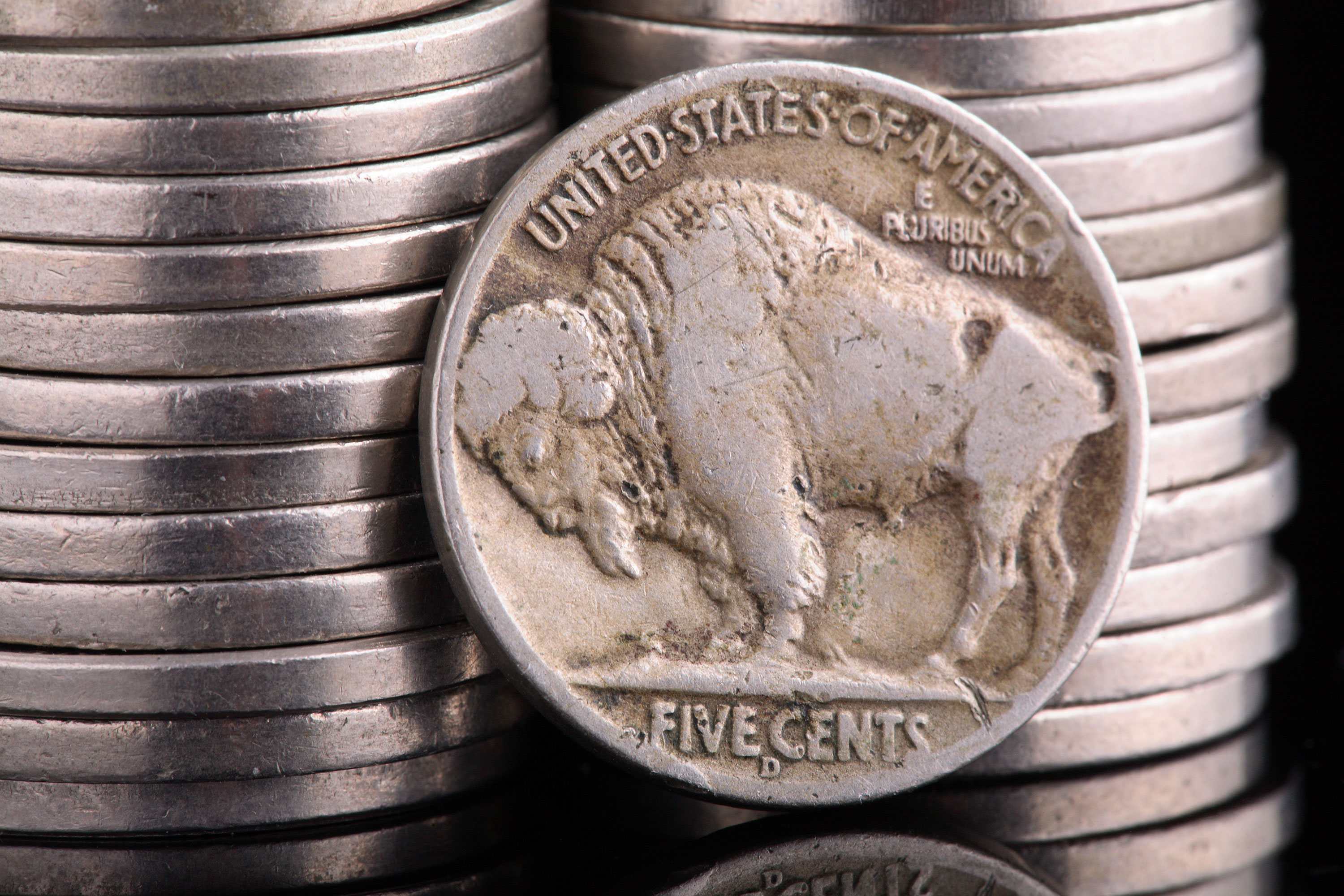The image is a detailed photograph featuring a close-up view of a well-preserved buffalo nickel, commonly known as a United States of America 5-cent piece. The coin, made of nickel-colored metal, prominently displays an engraved buffalo with its head facing left, featuring a lowered stance and a tuft of hair under its chin. The inscription "United States of America" arches across the top, with "E Pluribus Unum" and the denomination "five cents" engraved at the bottom, accompanied by the letter "D." The buffalo nickel appears slightly tarnished with a brownish hue around the top inscription but is otherwise in good condition with clear details. In the background, there are two to three stacks of similar nickels, their smooth edges creating a silver, metallic backdrop that towers in the zoomed-in perspective.